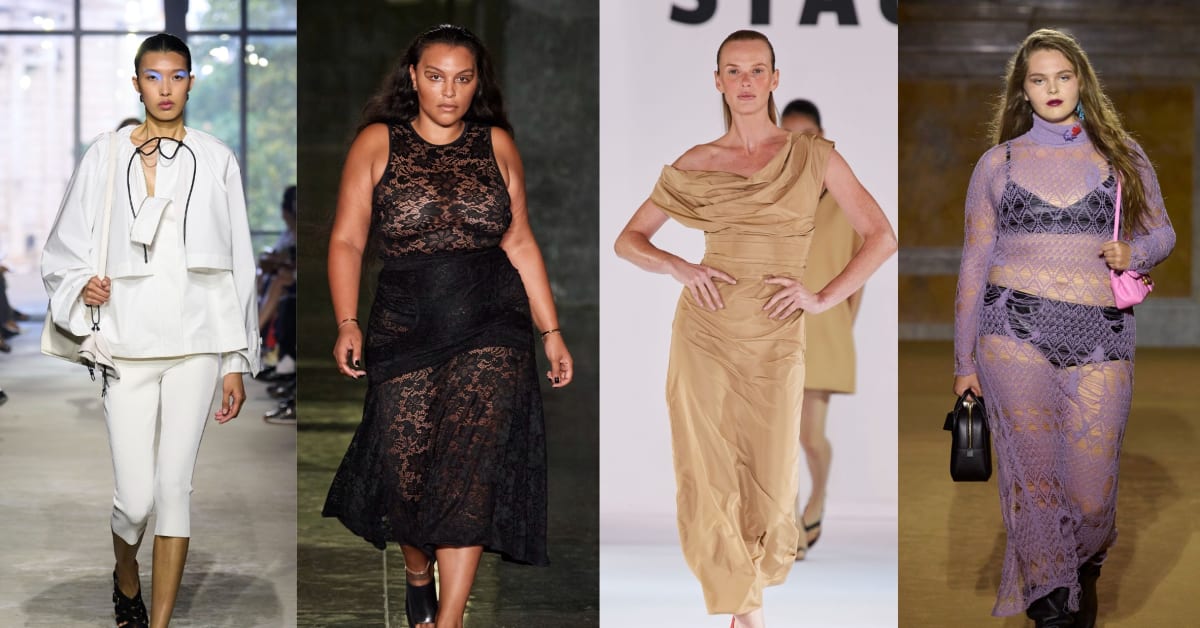This image collage showcases four models, each captured individually on a runway, portraying diverse styles and backgrounds. From left to right:

1. The first model, an Asian woman with very short black hair, is dressed entirely in white—donning a top with large sleeves and white pants. She carries a white bag on her right shoulder and sports striking blue eye makeup. She appears to be walking in front of large windows, which illuminate the scene with natural daylight.

2. The second model, a medium-sized woman with a darker complexion, is dressed in a distinctive black dress that features see-through elements at the top and bottom. Her long hair is let down naturally as she walks down the runway, emanating confidence.

3. The third model is a slender Caucasian woman in an elegant beige or bronze dress that provocatively slips off her right shoulder. Her hands are poised on her hips, adding to the gracefulness of her stance. She walks against a lighter background that complements her attire.

4. The final model, a curvier woman with long brown hair, stuns in a light lavender net dress. Beneath the semi-transparent fabric, she wears a dark bra and matching bottoms. She also wears black boots, and the background for her shot is a rich brown, adding depth to the image.

Each model embodies unique fashion sensibilities, with a mixture of textures, transparencies, and colors, set against distinctive yet complementary backdrops.